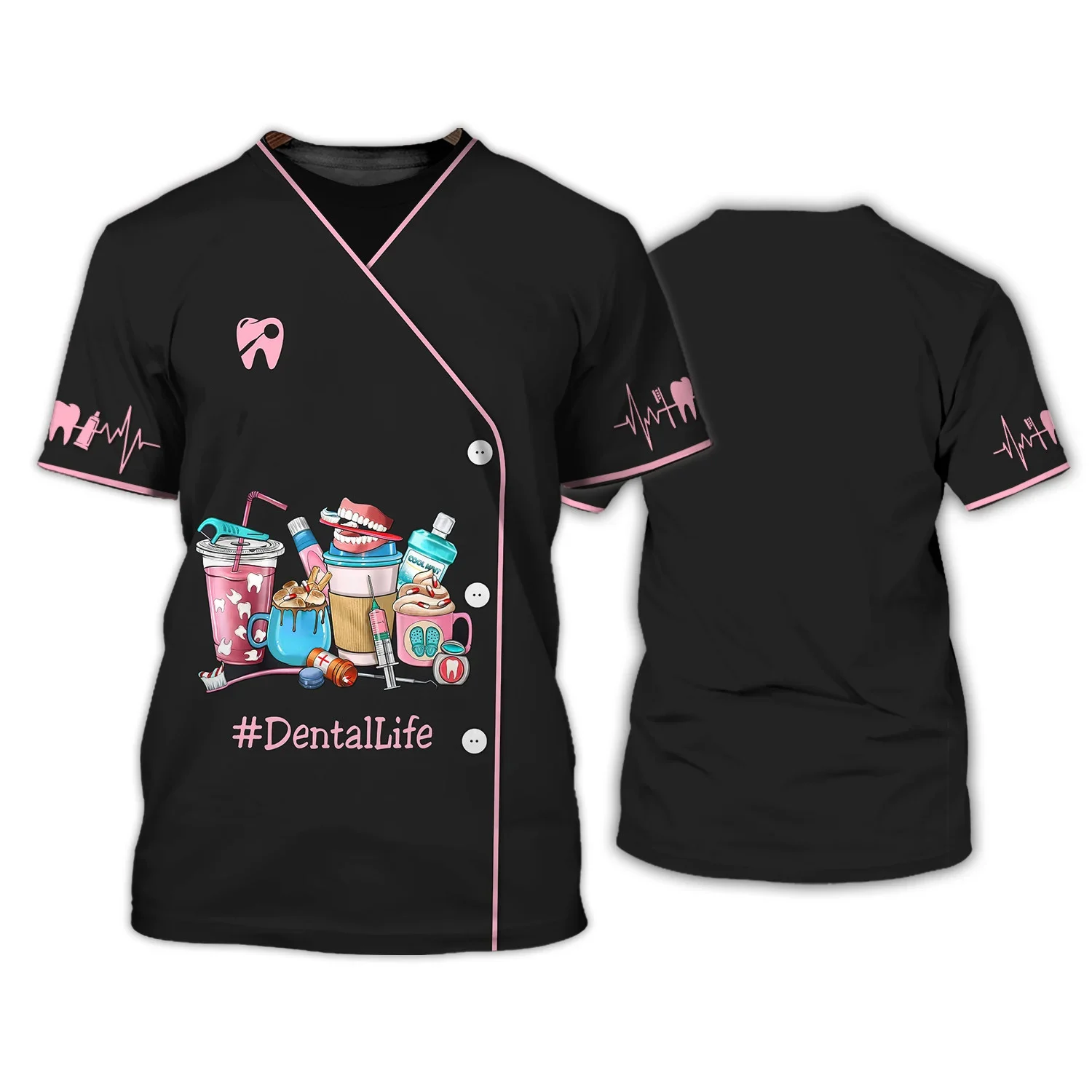This image is a color photograph, photoshopped to display both the front and back of a short-sleeved, black uniform top with pink trim, designed for dental professionals such as dental hygienists, assistants, or dentists. The front features a double-breasted button design, with three buttons running down the torso. The black fabric is adorned with numerous colorful, cartoonish dental-themed icons. Prominent images include a pink tooth, a dentist's flosser, a cup, a pair of chattering teeth, a syringe, a pill bottle, a soda can, floss stick, a toothbrush, and Listerine. Also depicted are non-dental items like chocolate, ice cream, a mug, and a cup of coffee. Below these illustrations, the text "#DentalLife" is prominently written in pink. The back of the shirt remains plain black.